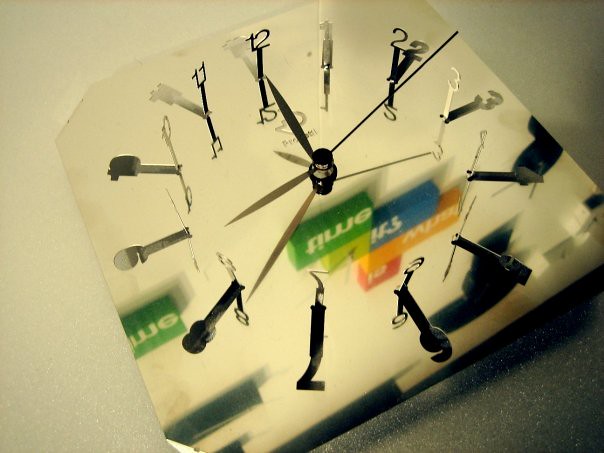The image depicts an unconventional clock constructed on a mirrored surface, creating a three-dimensional aesthetic. The clock is set on its backside, causing its numbers to rise vertically from black prongs, resembling a modern Stonehenge-style design. The numbers, which range from 1 to 12, cast visible shadows, contributing to a layered visual effect that can make reading the time challenging. The center features a screw anchoring the minute and hour hands, which point to the hour marker at 9 and the minute marker at 12, indicating 9 o'clock. The clock's background is white, while the numbers are predominantly black, with some white ones. Additionally, there are blocks of unreadable white text against green, blue, and orange backgrounds. The combined elements of multiple shades and repetitions add to the complexity of interpreting the clock's time and labels.